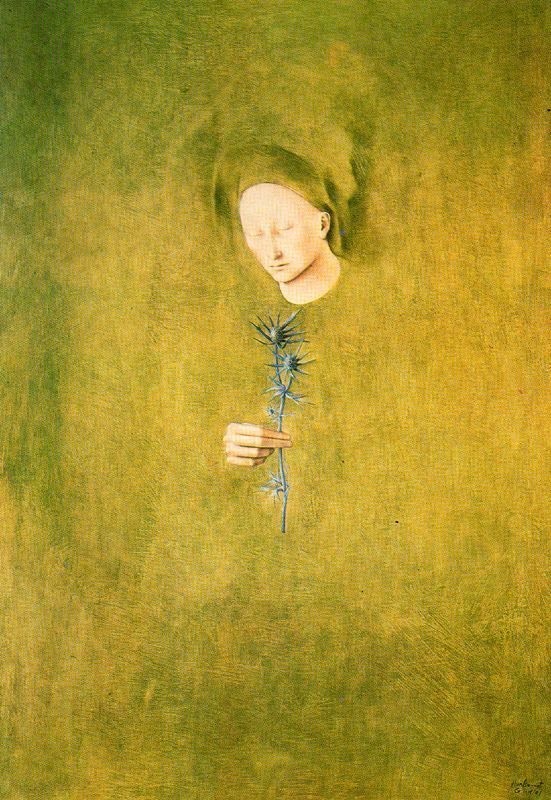This unique and striking painting features a minimalist composition set against a dual-shaded olive green background that subtly transitions from typical olive to a yellowish-green and back. Dominating the center is the face of an androgynous figure with a pale, almost white complexion, devoid of any hair and adorned with a head covering that mimics the surrounding background's greenish-yellow hues. With eyes closed and head tilted downward, the figure exudes a serene yet enigmatic presence. Emerging from the colored mist of the background, their hand extends delicately, two fingers carefully clutching thorny stems of decayed flowers that appear concrete-like, stripped of blossoms. These stems bear sharp, gray thorns arranged distinctly, with one stem showcasing eight thorns and the other with seven. The hand’s grip is gentle yet precise, suggesting a sense of fragility and reverence. Notably, the initials resembling "T" and "S" can be found at the bottom of this large-format artwork, adding a cryptic signature to this ethereal piece.